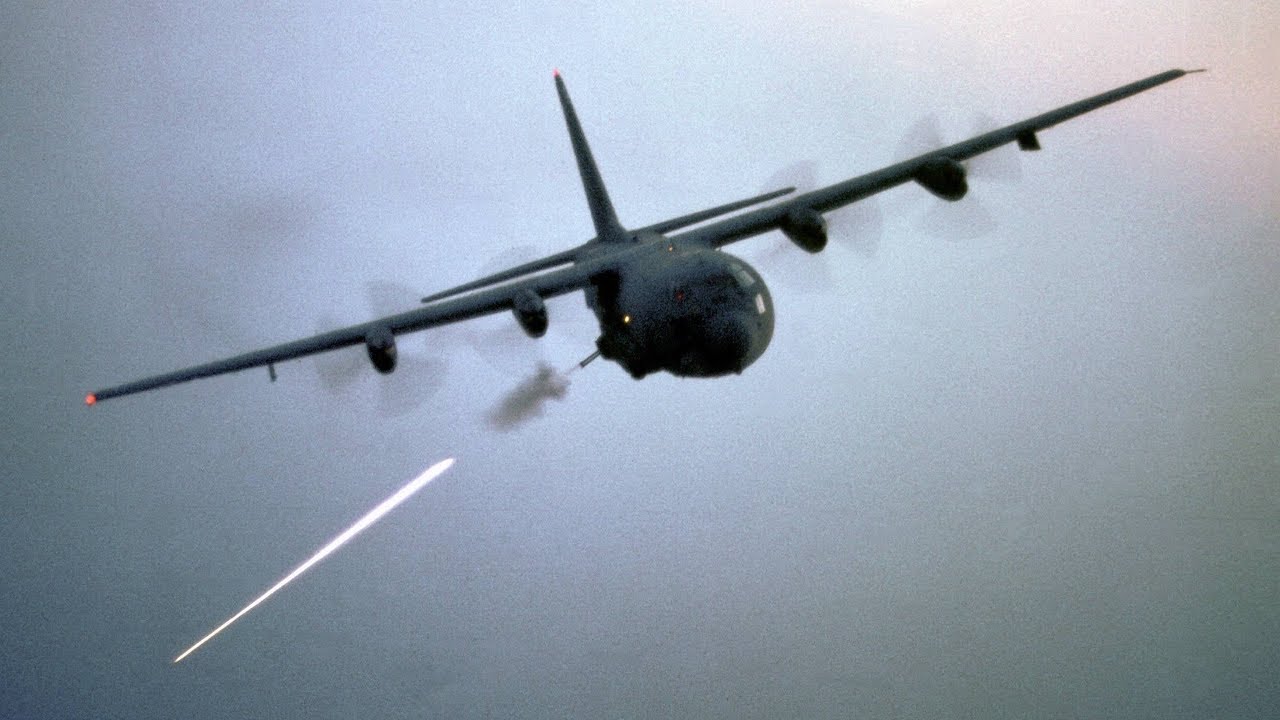This detailed photograph captures a military bomber airplane soaring through the sky. The plane, painted in dark military green, is equipped with four rapidly-spinning propellers, two on each wing, propelling it forward. The airplane, slightly tilted to the left with its right wing higher than the left, reveals an open side bay from which a machine gun protrudes. A soldier is visible, actively firing the weapon. The image vividly captures the muzzle flash, coupled with a stream of fire and a puff of smoke trailing from the gun, indicating that a projectile has just been fired. The sky behind the plane is gray, though it is unclear whether this is due to overcast conditions or if the image is in black-and-white, as the details are somewhat muted. At the front of the plane, the cockpit window is discernible. The plane's structure includes large, tall fenders at the back, pointing east and west, adding to its formidable appearance as it flies through the daytime sky.